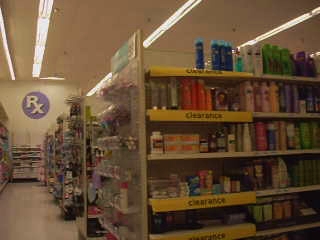This low-resolution, square-shaped photograph depicts the inside of a drugstore from one of the side aisles. Despite the blurriness, several details are discernible. The ceiling features two fluorescent lights shining white, lining the ceiling in parallel streaks. The focal point is a clearance section displayed on the first shelf to the right, prominently marked by a yellow banner on each level, reading "Clearance" in black text. The shelves in the foreground contain various products; on the upper levels are blue, white, and green shampoo bottles, while lower shelves hold orange bottles and possibly pink deodorants at the end caps. The image also shows numerous aisles stretching to the background, where a purple circle surrounds a white "RX" sign, suggesting the presence of a pharmacy section. The floor is white, extending back towards the wall of the store.